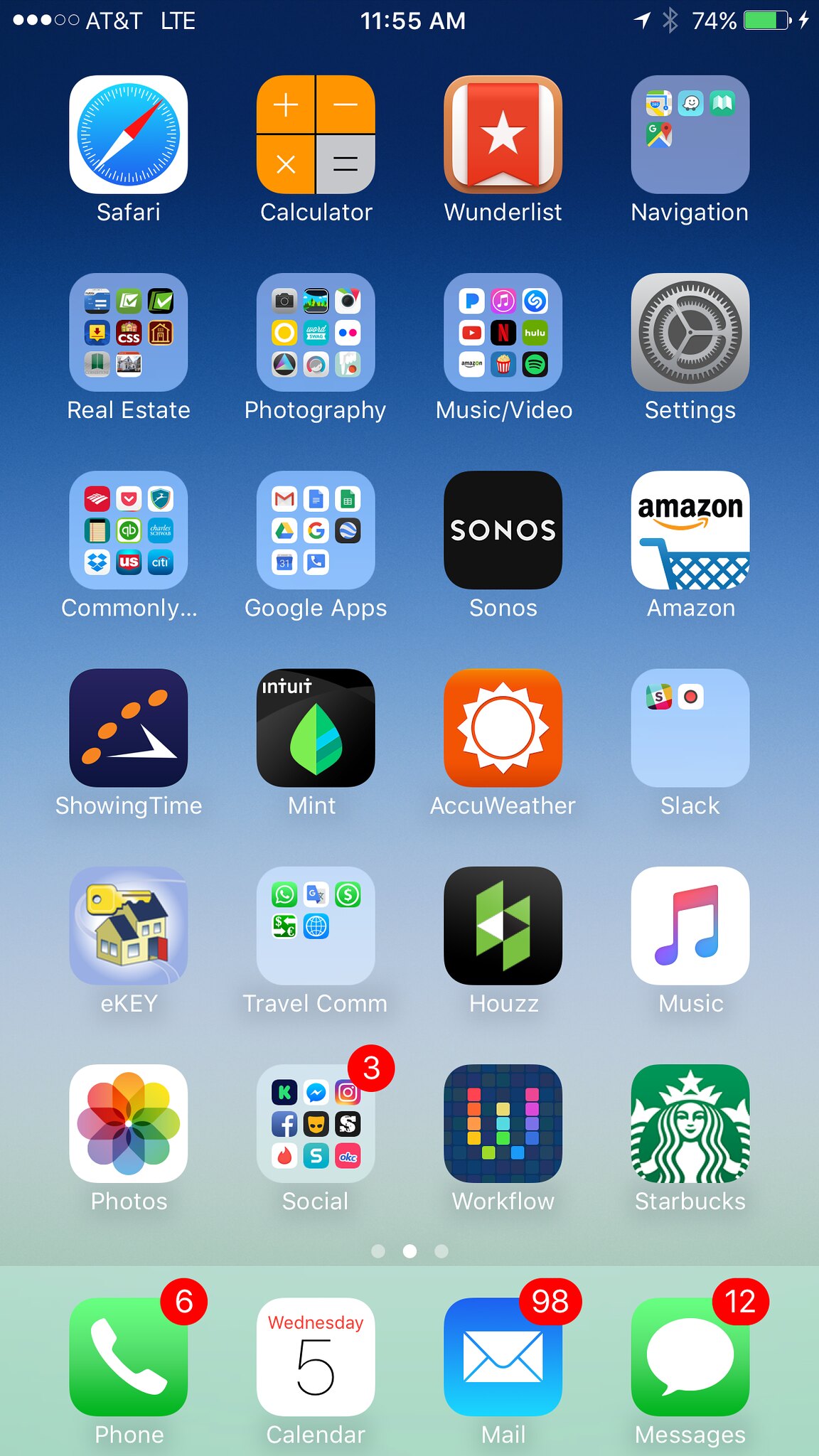Here is a detailed and cleaned-up caption for the screenshot of the phone:

---

A screenshot of a smartphone displaying the home screen. The status bar at the top shows the carrier as AT&T LTE, the time as 11:55 AM, and the battery at 74%. The home screen contains seven rows of app icons, organized in a grid layout with a multitude of folders and individual apps.

**Row 1:**
1. **Safari** - Icon with a white background and a blue compass featuring red and white dials.
2. **Calculator** - Icon with three yellow squares and one white square, displaying mathematical symbols: plus, minus, times, and equal.
3. **Wunderlist** - Icon with a white square, yellowish rim, red ribbon, and a white star.
4. **Navigation folder** - Contains Google Maps and three other navigation-related apps.

**Row 2:**
1. **Real Estate folder** - Contains eight apps related to real estate.
2. **Photography folder** - Contains nine apps associated with photography.
3. **Music/Video folder** - Contains nine apps, including Netflix, YouTube, Hulu, and Pandora.
4. **Settings** - Icon with a silver background and a gear symbol.

**Row 3:**
1. **Commonly Used folder** - Presumably contains nine frequently used apps, including Dropbox.
2. **Google Apps folder** - Contains eight apps, with Gmail in the top left and Google Chrome in the middle.
3. **Sonos** - Icon with a black background and white letters spelling S-O-N-O-S.
4. **Amazon** - Icon with "Amazon" in black text on a white background, featuring a blue shopping cart and a small arrow resembling a smile.

**Row 4:**
1. **Showing Time** - Dark blue icon with four yellow dots and a clock dial.
2. **Mint** - Black background with a green leaf and "Intuit" written on it.
3. **AccuWeather** - Orange background with a white sun symbol.
4. **Slack folder** - Contains two apps related to Slack.

**Row 5:**
1. **eKey** - Icon with a house and a key above it.
2. **Travelcom folder** - Contains five apps related to travel, including one with a dollar sign.
3. **Houzz** - Black background with green geometric shapes spelling "HOUZZ."
4. **Music** - White background with a dual-colored, pink and blue, musical symbol.

**Row 6:**
1. **Photos** - Icon with a colorful flower.
2. **Social folder** - Contains nine social media apps, with one displaying three notifications.
3. **Workflow** - Icon with a colorful digital "W."
4. **Starbucks** - Green background featuring the Starbucks siren with a crown and fish fin-like arms.

**Row 7:**
1. **Phone** - Green background with a white phone icon, showing six notifications.
2. **Calendar** - White background indicating "Wednesday, 5."
3. **Mail** - Blue background with a white envelope, showing 98 notifications.
4. **Messages** - Green background with a white chat bubble, showing 12 notifications.

---

This caption provides a detailed, clear description of the phone's home screen and the icons present on it, making it easy to visualize.